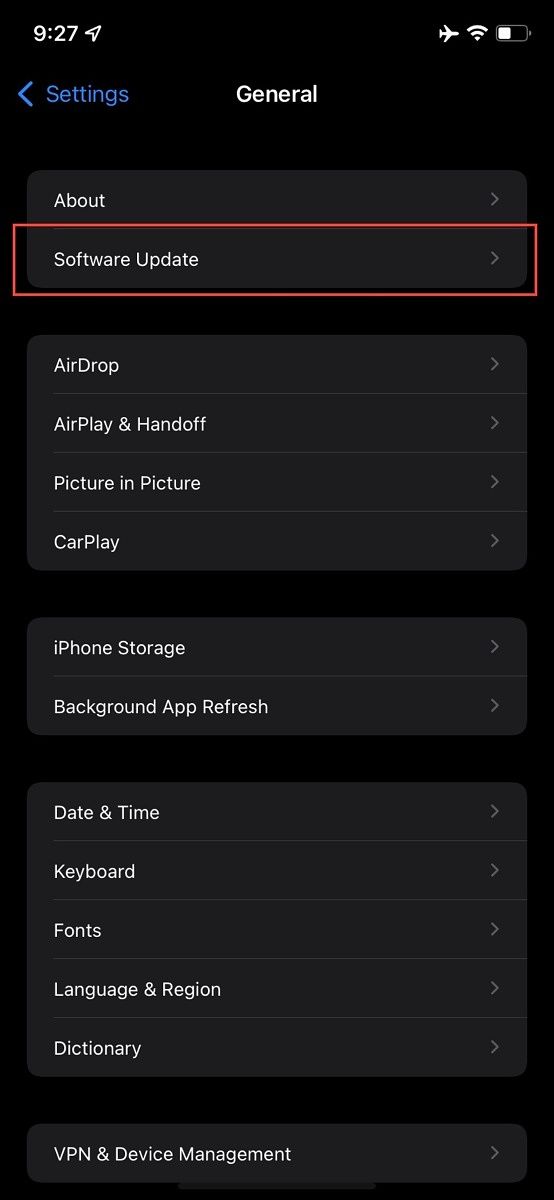The screenshot from a smartphone in dark mode has a black background, highlighting elements in white and blue fonts. The upper right corner displays the battery indicator, approximately half charged, alongside the Wi-Fi and airplane mode icons. On the upper left side, the time is shown as 9:27, though AM or PM is not specified. Below the time, "Settings" is written in blue with a left-pointing arrow beside it.

Centrally at the top, "General" is prominently displayed in white font. The remainder of the screen lists various menu items in white font, each with a right-pointing arrow indicating they are clickable for more options:
1. About
2. Software Update - highlighted with a thin red rectangle.
3. AirDrop, AirPlay, and Handoff
4. Picture in Picture
5. CarPlay
6. iPhone Storage
7. Background App Refresh

Further down, an additional section lists:
1. Date & Time
2. Keyboard
3. Fonts
4. Language & Region
5. Dictionary
6. VPN & Device Management

Each item on the list has a right-pointing arrow, indicating available submenus for further settings.